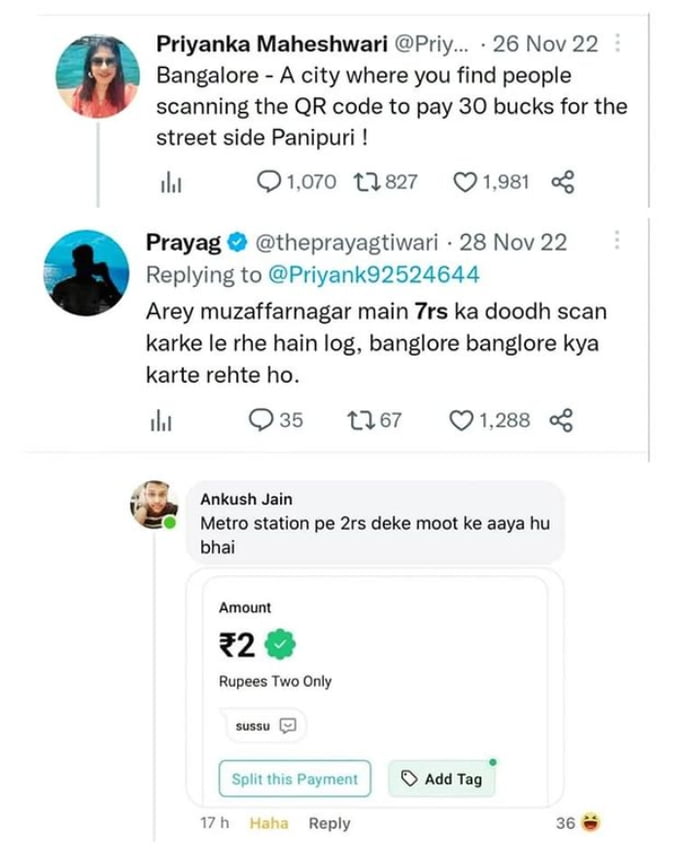**Caption**: 

In a vibrant Twitter/X post dated November 26, 2022, user Priyanka Maheshwari (@priyankamaheshwari) shares a moment in Bangalore, providing a modern snapshot of the city's street food culture. The image features Priyanka, a woman with long brown hair, dressed in a coral pink shirt, standing against the backdrop of an inviting, deep blue body of water. Her tweet captures the essence of urban life: "Bangalore, a city where you find people scanning the QR to pay 30 bucks for street-side pani puri."

The conversation thread includes a diverse group of users. One notable reply comes from Priya Yag (@prayag), who has a blue verified check mark. His profile image depicts him in silhouette, standing before a large, illuminated aquarium. However, his response is in a language unreadable to the user. Additionally, Ankush Jain (@ankushjain) participates in the thread, indicated by a green dot showing he is online. His profile hints at involvement with a metro station and suggests he has transferred money, labeled as "PE-2RS."

Overall, the image and accompanying text reflect the blend of traditional culture and cutting-edge technology in contemporary Indian urban life.